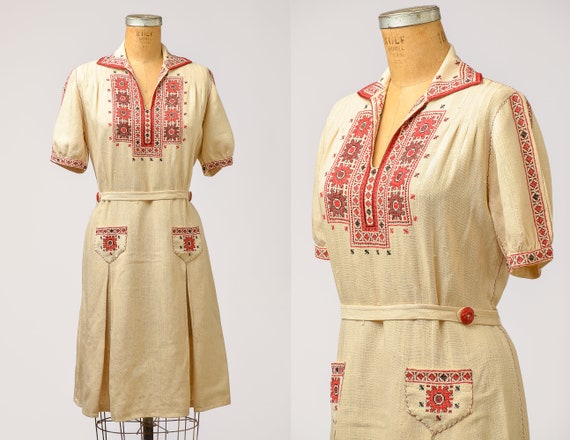The image displays two side-by-side photos of a dress on a headless, armless mannequin, allowing for a clear focus on the garment. The dress is crafted from what appears to be linen or cotton, featuring a mid-calf length peasant style with a belt. The dress has a V-neck with an open collar in a creamy, light-yellow hue. The short sleeves extend about halfway down the arm. Embroidered patterns of red, pink, and purple flowers adorn the neckline, sleeves, and two small pockets located near the lower part of the dress. The intricate floral embroidery around the V-neck, sleeves, and pockets gives the dress a charming, country aesthetic. The overall color of the dress is a subtle beige, enhanced with red buttons down the front.